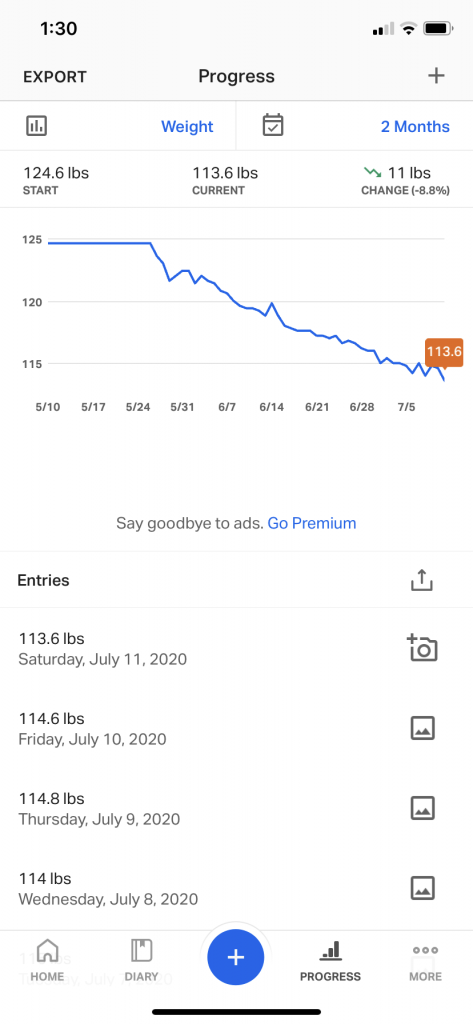This image showcases a screenshot of a weight loss or fitness tracking app on a mobile device, displayed in a portrait orientation. The screenshot, approximately three times as tall as it is wide, features a predominantly white background. At the top, there is a gray header bar displaying a time of 1:30, an "Export Progress" label, nearly full battery icon, and indicators for network connection and WiFi strength.

Beneath the header, two sections are separated by a vertical divider: "Weight" accompanied by a chart icon, and "Month," displaying data for two months. Further down, detailed weight information is presented: a starting weight of 124.6 lbs, a current weight of 113.6 lbs, and a weight change of -11 lbs, indicating an 8.8% decrease.

A graph below this information charts weight changes over time, with the horizontal axis ranging from 5'10 to 7'5 and the vertical axis from 1'15 to 1'25. The graph depicts a downward trend, culminating at 113.6 lbs. 

Following a divider line, additional tabs are present, including an "Entries" tab with an upload button. This section lists individual entries by date, specifically July 11th, July 10th, July 9th, and July 8th.